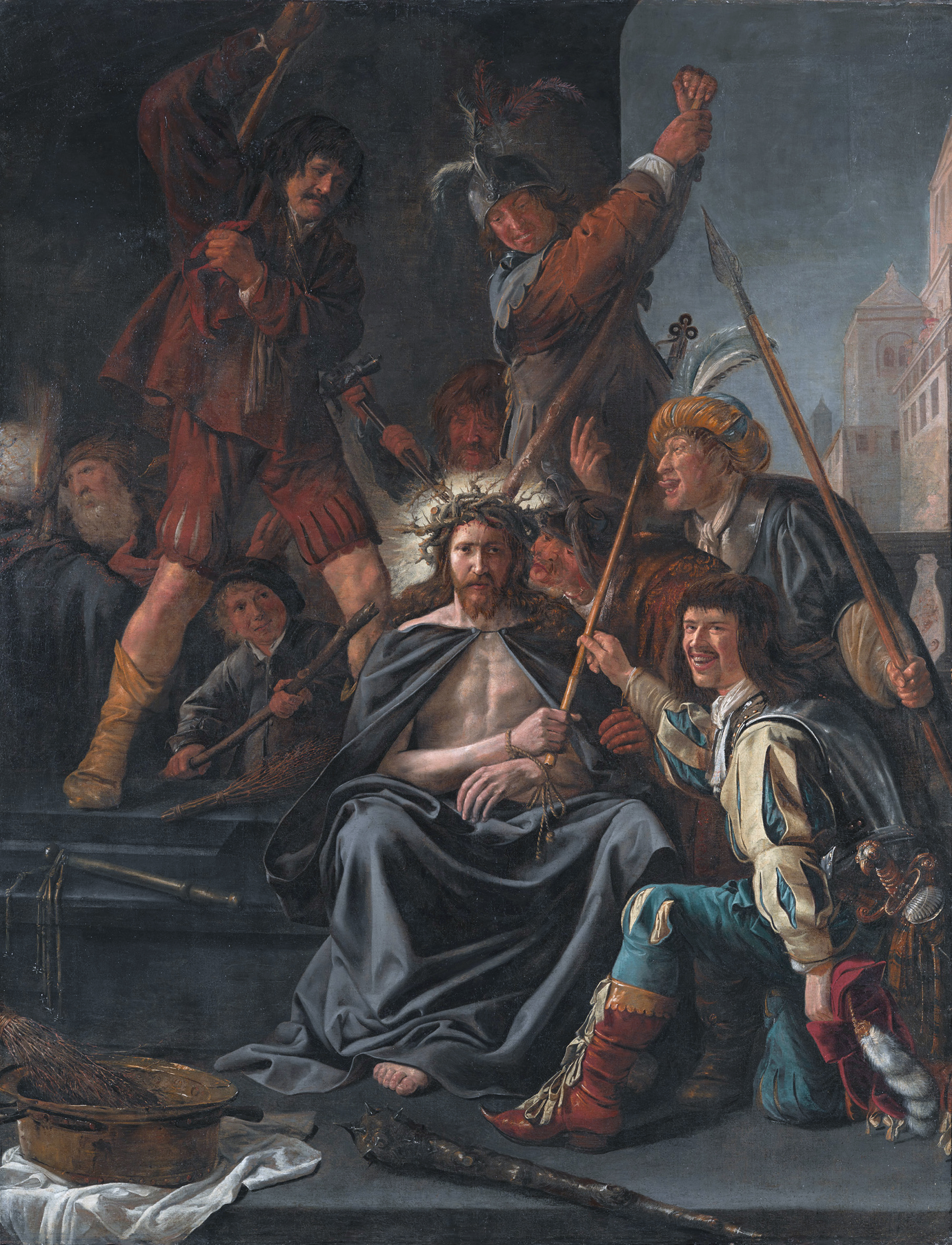The image is a detailed and realistic artwork depicting a scene from the crucifixion narrative, where Jesus Christ, adorned with a crown of thorns, is being mocked and tormented. Central to the composition, Jesus sits shirtless with a blue robe draped over his legs, holding a staff with a cross at the top. His curly black hair and long beard are evident. He is encircled by seven men in medieval attire, including white and silver armor, blue pants, red boots, and red coats, some of whom are seen laughing and jeering at him. One man to Jesus’ right is particularly notable, looking off to the left with a smile. The ground beneath them appears to be gray stone, and towards the lower left, there is a pot placed on a white cloth. A weapon, possibly a spiked club, lies on the ground near the men. Behind Jesus, additional figures are visible, some looking menacing with raised arms and weapons. The background features medium to dark gray skies and beige stone buildings, further emphasizing the somber and ominous atmosphere of the scene.